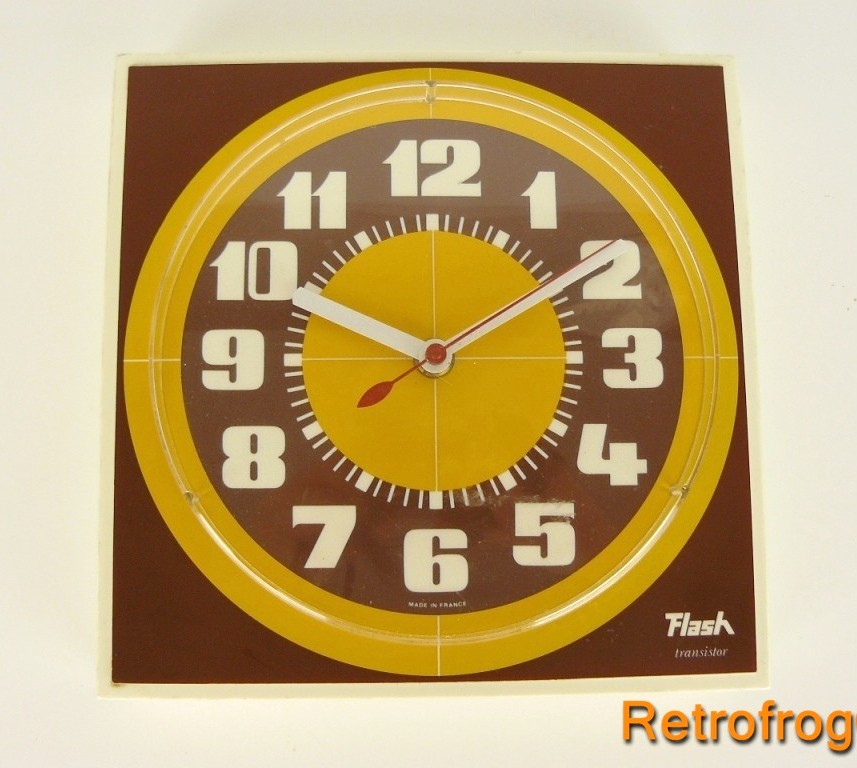The image displays a clock with distinctive features. The clock face is bordered in brown, with the bottom edge illuminated by a flash. Centrally, there is a prominent yellow circular shape, repeatedly framed by smaller concentric yellow circles. These yellow circles are intersected by a prominent line running through the middle. The clock hands are positioned such that the hour hand points to ten, the minute hand to two, and the second hand also to two. The clock face is encircled by dash marks indicating the hours. To the far left of the clock, the border is white. At the bottom of the image, text reads "Made in France."